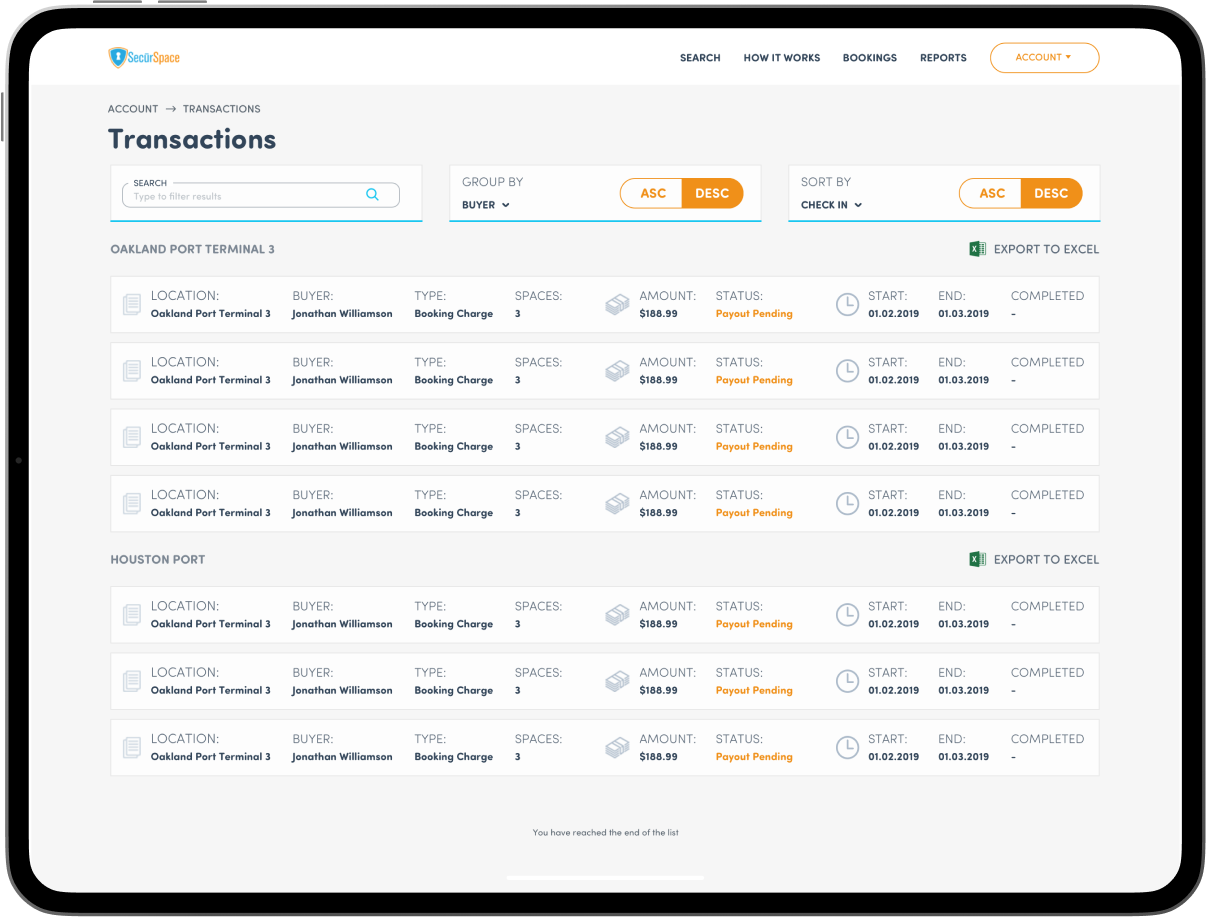This screenshot captures a detailed interface of an application viewed on a tablet with a landscape orientation. The screen's upper left corner prominently features the logo "SECUR-SPACE" with an umlaut over the 'U'; "SECUR" is colored blue, while "SPACE" is orange. In the upper right, a navigation menu includes options such as "Search," "How It Works," "Booking," "Reports," and an "Accounts" dropdown button, all displayed in an orange font and outlined in orange.

Directly below, a gray background section labeled "Transactions" contains a search bar prompting users to "Type to filter results." Adjacent to the search bar, a dropdown menu labeled "Group By" displays "Buyer" as the default option. Further right, two buttons, "ASC" (white with orange font) and "DESC" (orange with white font), offer sorting options. Another dropdown menu labeled "Sort By Check-In" provides additional sorting functionality.

The primary content area lists seven lines of transaction data, with the header identifying the location as "Oakland Port Terminal 3." Detailed fields for a specific transaction include: 
- Location: "Oakland Port Terminal 3"
- Buyer: "Jonathan Williams"
- Type: "Booking Charge"
- Spaces: 3
- Amount: "$188.99"
- Status: "Payout Pending"
- Start Date: "01.02.2019"
- End Date: "01.03.2019"
- Completion Status: "Completed"

An "Export to Excel" link is available above the transaction details for data export purposes.